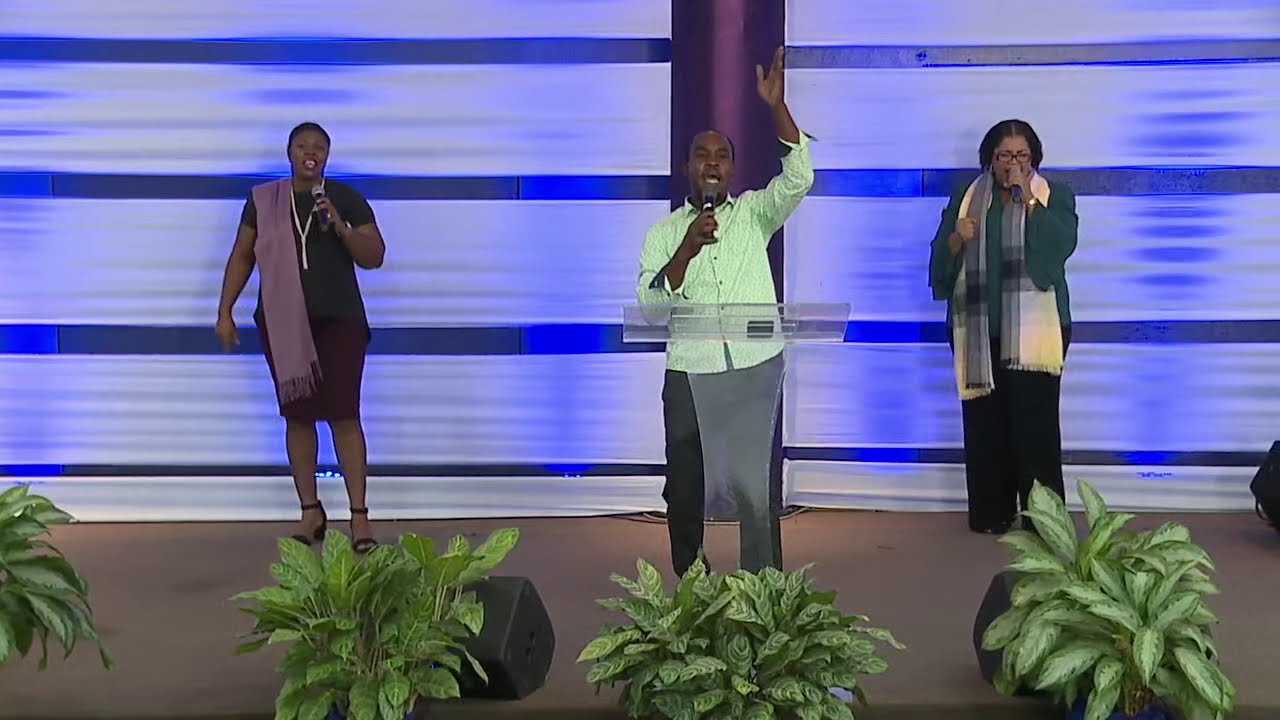The photograph depicts a scene from what appears to be a large church or similar indoor setting. At the center stands an African American man, dressed in a light mint green long-sleeved shirt with collars and black pants, featuring an unusual gray drape over them. He is holding a microphone up to his mouth with one hand while his other hand is raised high in the air. Flanking him on both sides are two African American women, similarly holding microphones, suggesting they are singing. 

The woman to his left is dressed in a black skirt, a black top, and a dull lavender scarf, while the woman to his right wears a dark forest green top with black pants and a yellowish scarf. In the foreground of the stage, there are four green leafy plants in pots, strategically placed to conceal black stereo sound systems. Behind the group, the backdrop consists of strips of various fabrics laid horizontally, featuring colors such as light green, green, light blue, dark blue, light purple, dark purple, lime, burgundy, and violet. The setting appears to have been captured indoors, with no visible religious iconography, but the arrangement and attire suggest a church service or concert.